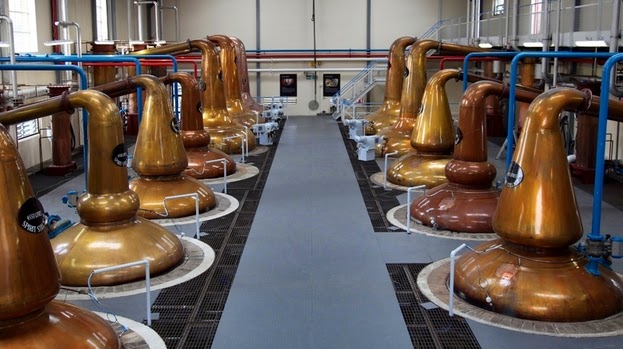This photograph captures the interior of an expansive factory, specifically a distillery where alcohol is produced. The focal point is a long, gray flooring that extends from the top to the bottom of the image, running through the entire length of the factory. On this floor are strategically placed black vents, presumed to be exhausts, designed with small perforations for efficiency.

Flanking the central pathway are rows of large vats, primarily golden-bronze in color but varying slightly in hue. These vats, totaling twelve, are used for the processing and storage of liquids. The distribution is uneven, with seven vats situated on the left side and five on the right side. These vats are interconnected with a complex network of metallic tubing that traverses the facility, highlighting the intricate infrastructure needed for the distillation process.

Additionally, blue poles are attached to some parts of the equipment, connecting various components and possibly facilitating the movement of materials or stabilizing structures. In the background, a stark white wall decorated with black lines stands out against the gray side walls, which house several windows, casting natural light into the workspace. The meticulous arrangement and connectivity of all these elements underscore the sophisticated operations within this distillery.